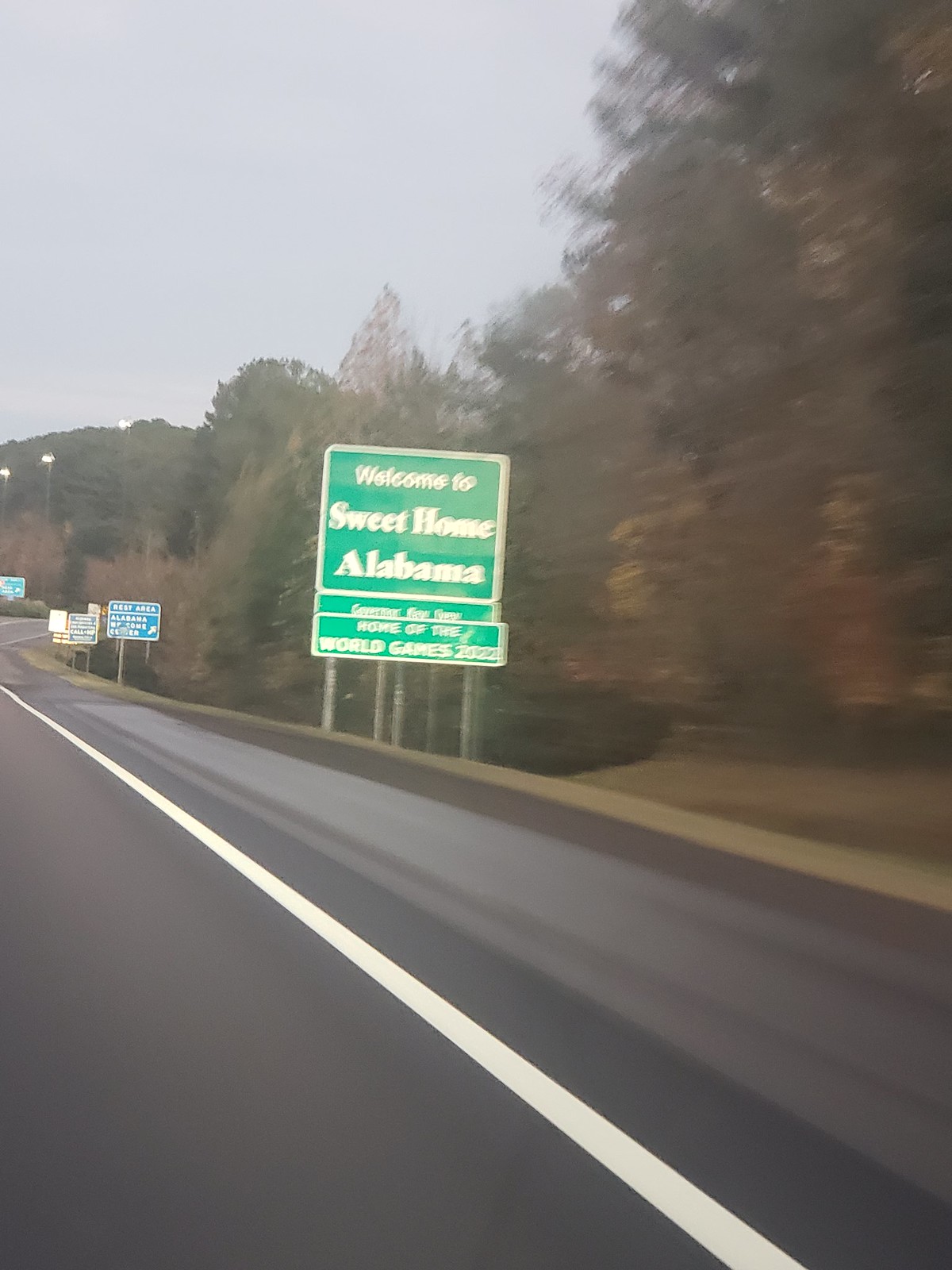This photo, taken from a moving vehicle, captures a "Welcome to Sweet Home Alabama" road sign situated a short distance ahead. The square green sign features a thin white border with the welcoming message in white letters. Below it, there is an unreadable smaller rectangular sign, and beneath that, a larger rectangular sign also obscured due to the photo's motion-induced blur. On the right side of the freeway, the roadside is bordered by a dense line of trees. Further in the background to the right, a blue rectangular road sign with white text and a small white border indicates the presence of a rest area.